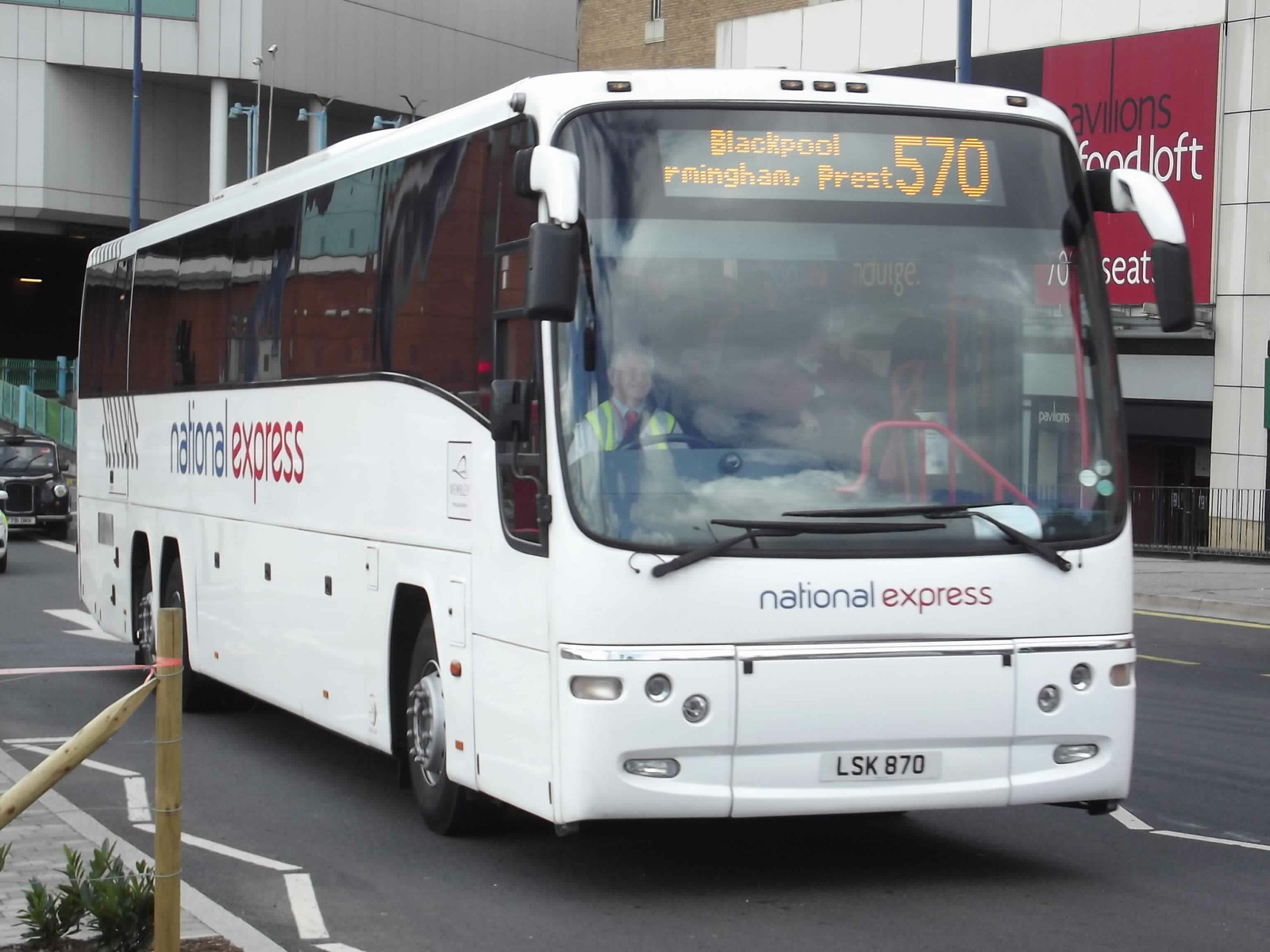The photograph features a large, white long-distance bus prominently labeled with "National Express" on both its side and front. The word "National" is in blue while "Express" is in red. Above the windshield, a digital display in orange reads "Blackpool Birmingham PREST 570," though the word "Birmingham" is partially obscured. The bus is positioned on a paved city street, facing slightly to the right, revealing both its right side and front. In the background, there's a large gray building, likely a bus terminal, with cars and other details visible behind the bus. The bus driver, visible through the windshield, is dressed professionally in a suit and tie with a reflective yellow vest, and he appears to have white hair. The image captures the bus seemingly preparing to depart from the terminal.